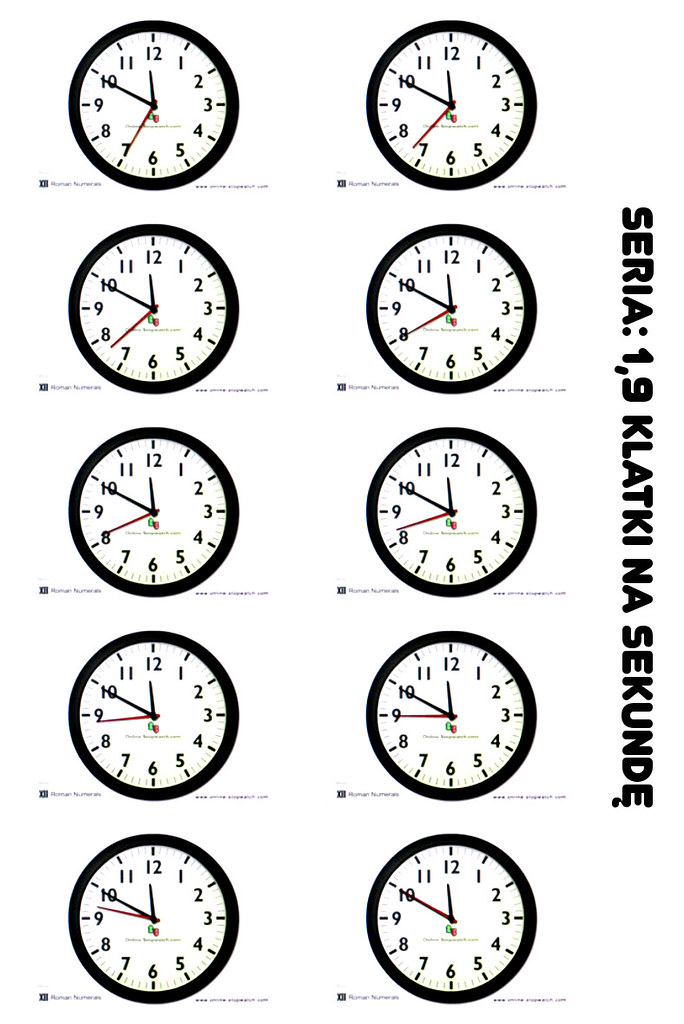The image features ten clip-art-style clocks arranged in five rows of two against a plain white background. Each clock is black-rimmed with a basic white face, displaying traditional black numerals from 1 to 12 and lighter black minute marks. All clocks show the time as 11:50, but the red second hand is positioned differently on each clock, indicating a progression of seconds from top left to bottom right. To the right of the clocks, in dark bold uppercase letters, is the text "S-E-R-I-A-1-9-K-L-A-T-K-I-N-A-S-E-K-U-N-D-E" running vertically down the side. Additionally, there are words appearing beneath each clock, although specific details about these words are not provided. The image concludes with the phrase "Thanks for watching!" repeated twice.